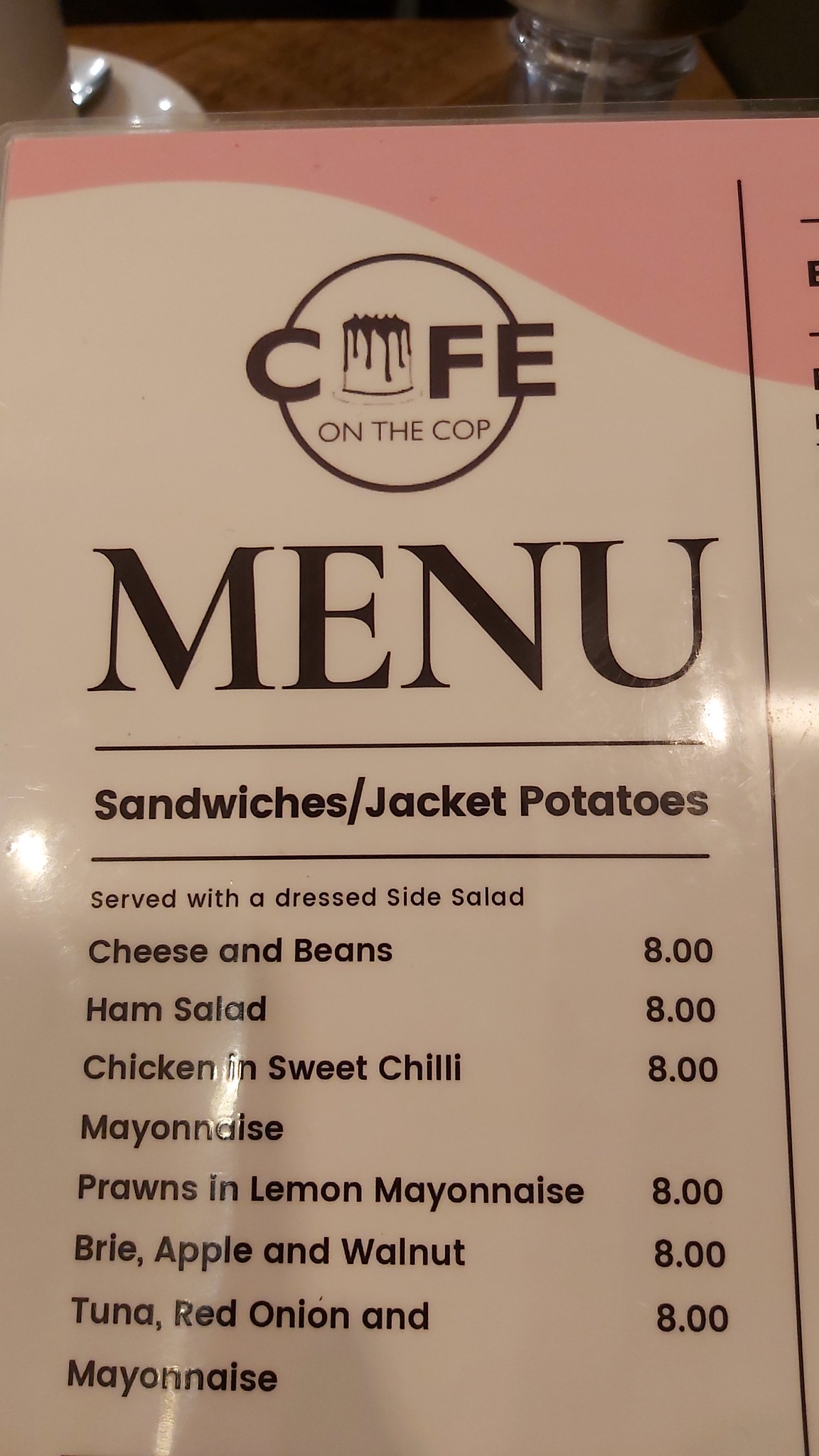This photograph captures a detailed view of a laminated menu page set against a wooden parquet table background. In the upper left corner, partially out of frame, a tea saucer with a teacup rests beside what appears to be a glass of water, hinting at a recently occupied table. The menu itself is stark white, dominated at the top by a prominent black circle featuring a stylized graphic of a cake, dripping with chocolate or dark frosting. Centered within the circle is the letter 'C', followed by the letters 'F' and 'E', strategically placed to spell 'Café' when read together.

Directly beneath this, in bold black font, the word 'Menu' is prominently displayed, underlined for emphasis. Further down, headings divide the offerings: 'Sandwiches / Jacket Potatoes' followed by another underline, leading into the specifications 'served with a dressed side salad'. The menu lists various sandwich and jacket potato options, each priced at eight dollars: Cheese and Beans, Ham Salad, Chicken and Sweet Chili, Prawns and Lemon Mayonnaise, Brie and Apple and Walnut, and Tuna and Red Onion with Mayonnaise. Notably, a listing for 'Mayonnaise' lacks an accompanying price. The detailed layout suggests a welcoming café environment, offering a variety of hearty meal options.